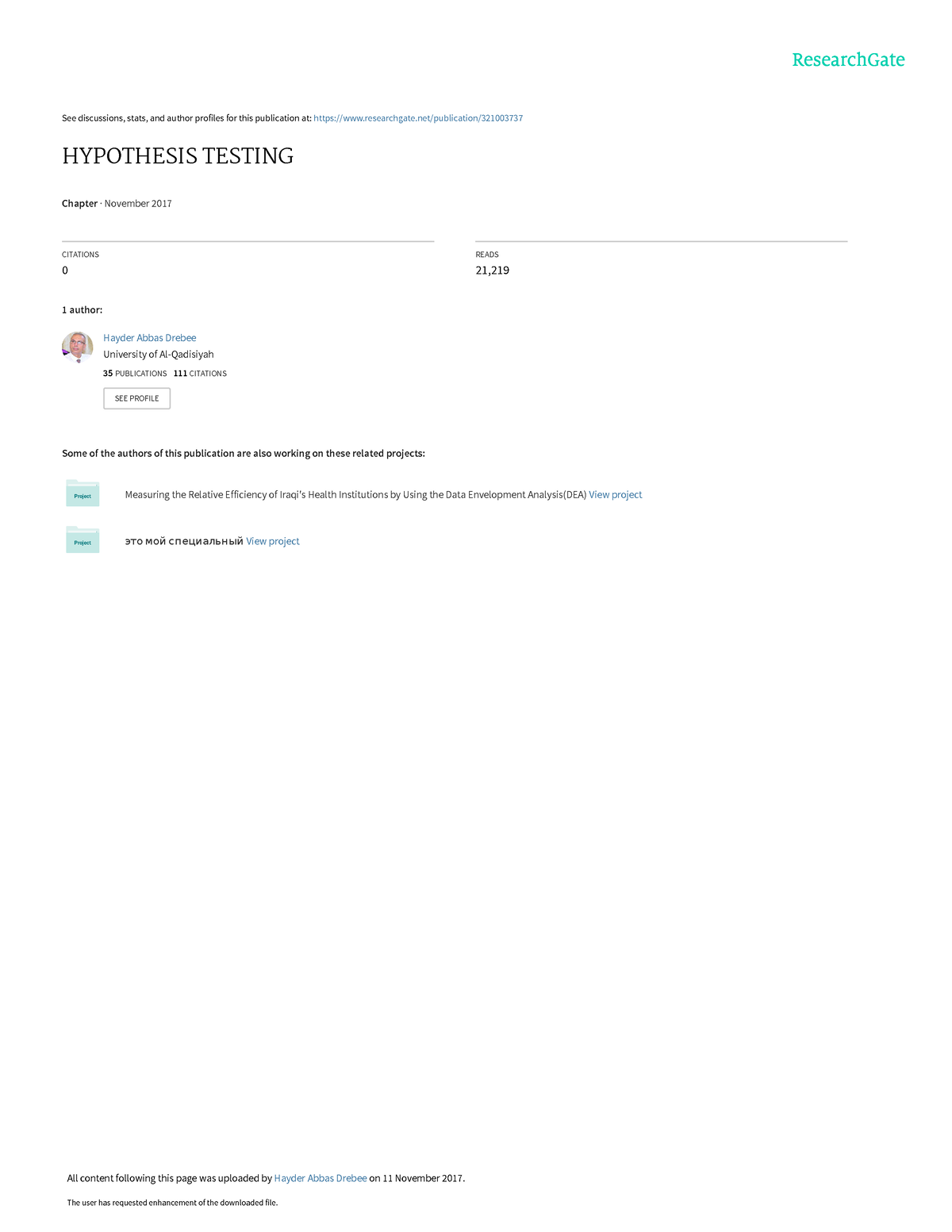The image appears to be a screenshot from a website with a white background and black text, featuring several elements in blue and green. At the top right corner, the website is identified as ResearchGate. On the left-hand side above the heading, there is a line in an extremely small font that concludes with blue text, indicating a clickable link.

The main heading, left-justified in capital letters, reads "HYPOTHESIS TESTING." Below this is a chapter selected from a drop-down text box. Following this are two light gray lines, with content written beneath them too small to decipher. Then, a section in bold text appears, accompanied by a tiny round profile picture, presumably of a researcher, with their name next to the picture in blue text, which is also too small to read.

Underneath, there are two lines of black text, followed by a button. Near the bottom, a black bold line is visible, followed by two buttons with associated information. Each piece of information ends with a blue clickable link. Finally, there's minuscule writing at the very bottom of the page.